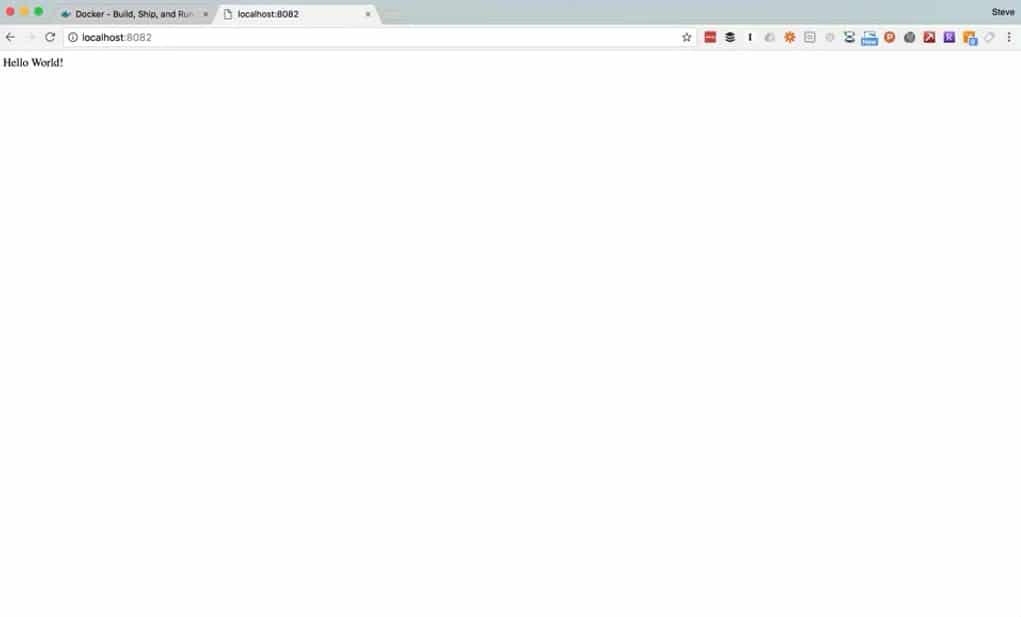This screenshot captures a browser window on a Mac computer, identifiable by the red, yellow, and green circles on the top-left corner which are used to close, minimize, or maximize the browser. The URL displayed in the address bar is "localhost:8082," indicating a local server. The content of this page is minimal, featuring a single line of text: "Hello, World!" with an exclamation mark, centered on a blank white background.

Adjacent to this tab is another open tab labeled "Dockers," suggesting it could be related to Docker, a popular platform for developing, shipping, and running applications. The browser's bookmark bar is packed with around 15 to 20 bookmarks, including familiar icons such as settings, weather, and news (possibly CNN).

Overall, this image showcases a simple localhost page with minimal content, being displayed on a Mac's web browser with multiple utility bookmarks.